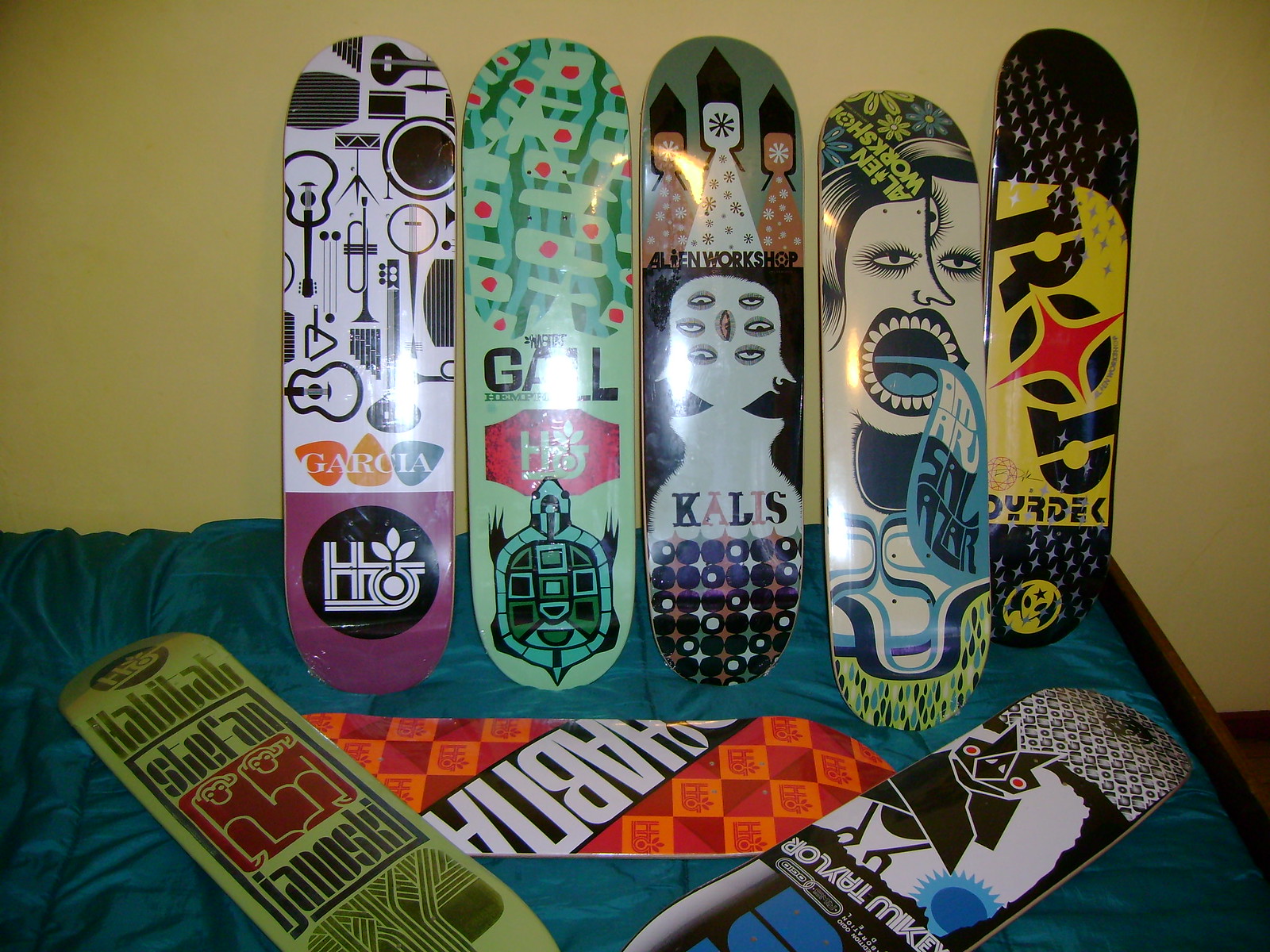In this detailed photograph, eight wheel-less skateboards with diverse designs are featured against a soft greenish-yellow wall and atop a bed with a blue blanket. The bed itself is constructed from dark brown wood. Five skateboards are leaning against the wall at the head of the bed, and three are laid flat on the blanket.

Starting from the left, the first skateboard has a white top adorned with musical instruments, a purple bottom featuring a circle with a letter "H" and a plant. Next to it, the second skateboard has a primarily green design with red dots at the top, a turtle at the bottom, and lettering in the middle that reads "G-A-L-L." 

The third skateboard over has a unique image of two faces on a single head, each looking in opposite directions, with six eyeballs in the middle, and the text "K-A-L-I-S" written on it. To its right, the fourth skateboard shows a female figure with an open mouth from which water seems to flow, and lettering that appears to say "A-M-A-R-S-A-L-A-Z-A-R."

The fifth skateboard is primarily black with a yellow middle section and red-starred "O," spelling out "R-O-B."

On the bed, starting from the bottom left, an olive green skateboard features two monkeys on a red background. Nearby, an orange and red skateboard shows large white letters on a black diagonal stripe. Lastly, at the bottom right, another black skateboard boasts an illustration of an owl with a blue sun and the text "T-Y-L-E-R, Mikey."

The varied and vibrant designs of the skateboards, set against the aesthetic background, make this a captivating and detailed image.